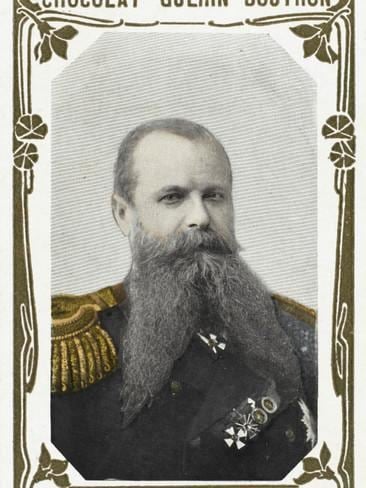The photograph captures a detailed portrait of an older man, likely from the 1800s, suggestive of a military figure such as a general. The man, approximately 50 years old, has a long beard divided into two distinct sections, the hair within his beard transitioning from dark gray at the roots to lighter gray towards the tips. His receding hairline reveals gray hair combed back smoothly. Dressed in a black or dark-colored military uniform, it's adorned with gold tassels on the right shoulder and various military medals and pins on the left breast. Gold buttons further embellish his attire. The background of the portrait consists of fine gray and white diagonal stripes, adding a subtle contrast to the image. Surrounding the photo is a brown border featuring a design reminiscent of leaves and twigs with scattered flowers, potentially greenish-gray in tint. At the top of the image, there is some partially cut-off text, likely in a similar grayish hue.